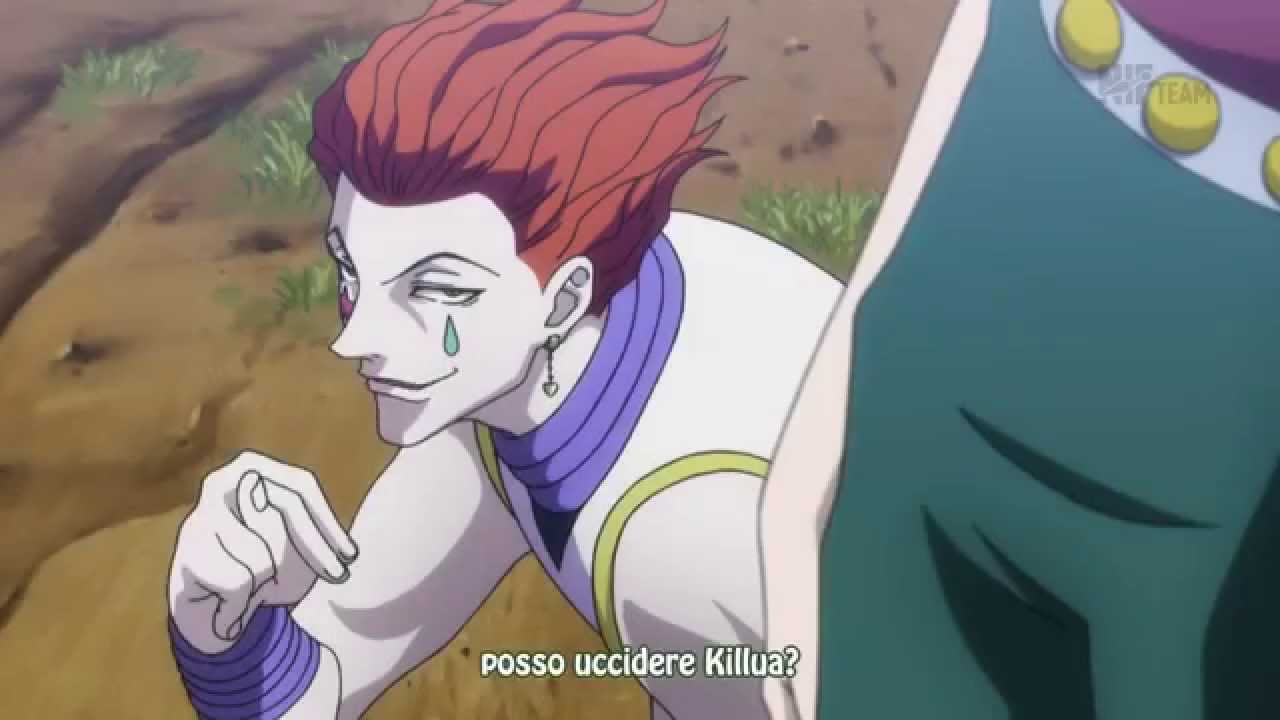The image is a still from an animated series featuring a character with a distinctive and flamboyant appearance. The character, likely male, has flaming bright red spiky hair brushed straight back, giving a wind-blown effect. His face is chalky white, almost clown-like, with dramatic dark-lined eyes and dark arched eyebrows. He has a green teardrop tattoo just below one eye, enhancing his sly and confident expression. A large hoop earring adorns his left ear, while his attire includes a white top with a high collar and purple trim, complemented by a cape or shawl with a purple lining and yellow circular details, secured by a gold clasp or brooch. The character’s hands are notably positioned with his thumb between his second and third fingers.

He appears to be in a crouched position, looking upward towards another character whose knee is partially visible. The scene is set against a blurred outdoor background with a dirt ground and sparse patches of grass, suggesting a barren or agricultural environment. Overlay text at the bottom reads "POSE FUSIDERE KILUA" with a question mark, indicating a subtitle in a non-English language. A partially faded logo in the top right corner seems to read "N-H-E TEAM".